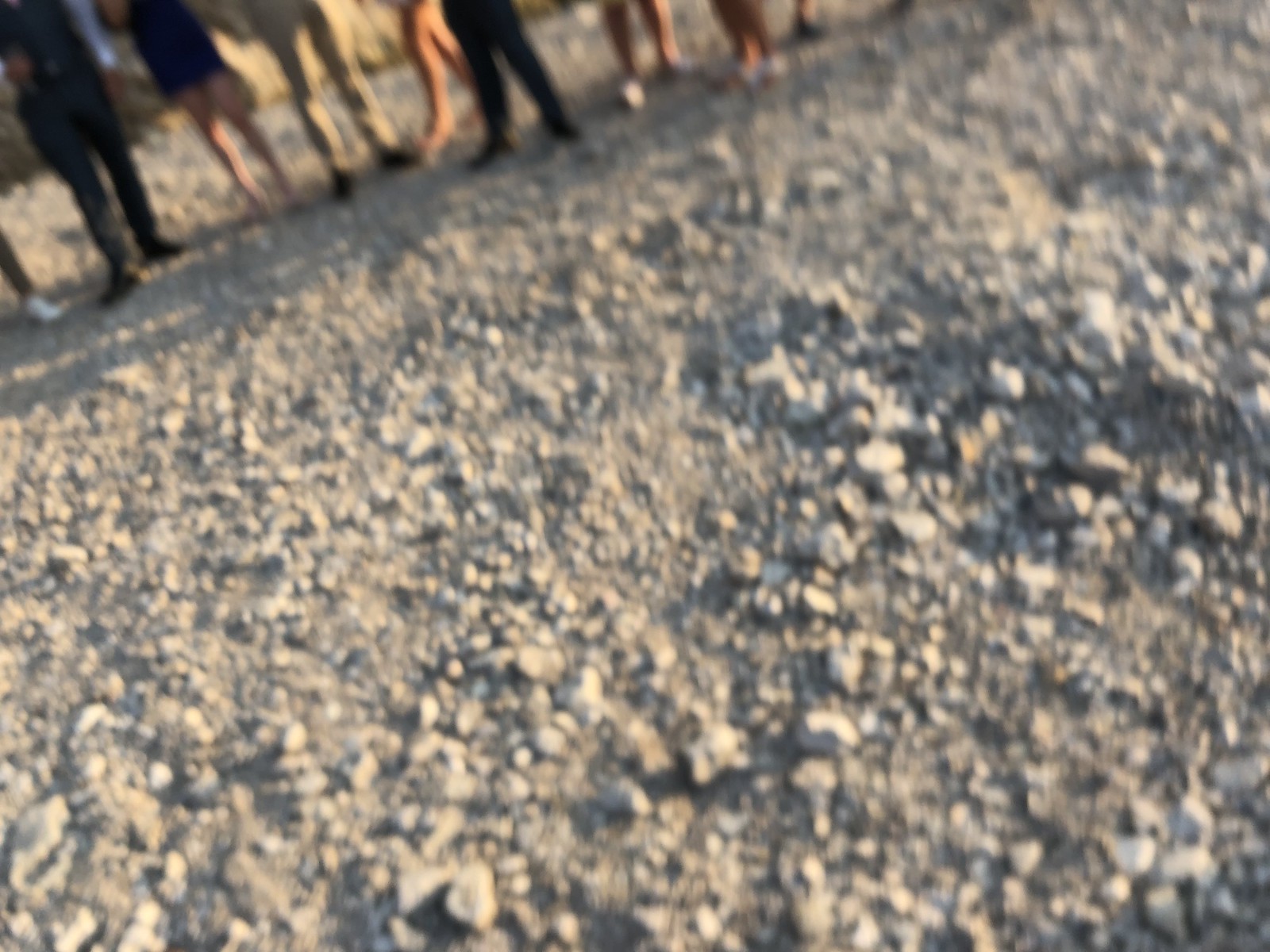This outdoor daytime photograph predominantly features a close-up view of variously sized pebbles and gravel, covering roughly 80% of the image. The gravel appears in different shades of gray, beige, and brown, slightly blurred to create a somewhat indistinct texture. In the upper left-hand corner, a line of people stands at a 45-degree angle. Only their legs and feet are visible: trousers and shorts of different colors, including dark pants, brown shorts, and khakis, as well as a mix of footwear. Shadows of their legs fall onto the ground, contributing to a sense of depth and dimension in the image. This overall scene gives the impression of an unintentional shot, perhaps taken when the photographer's camera inadvertently tilted downward.